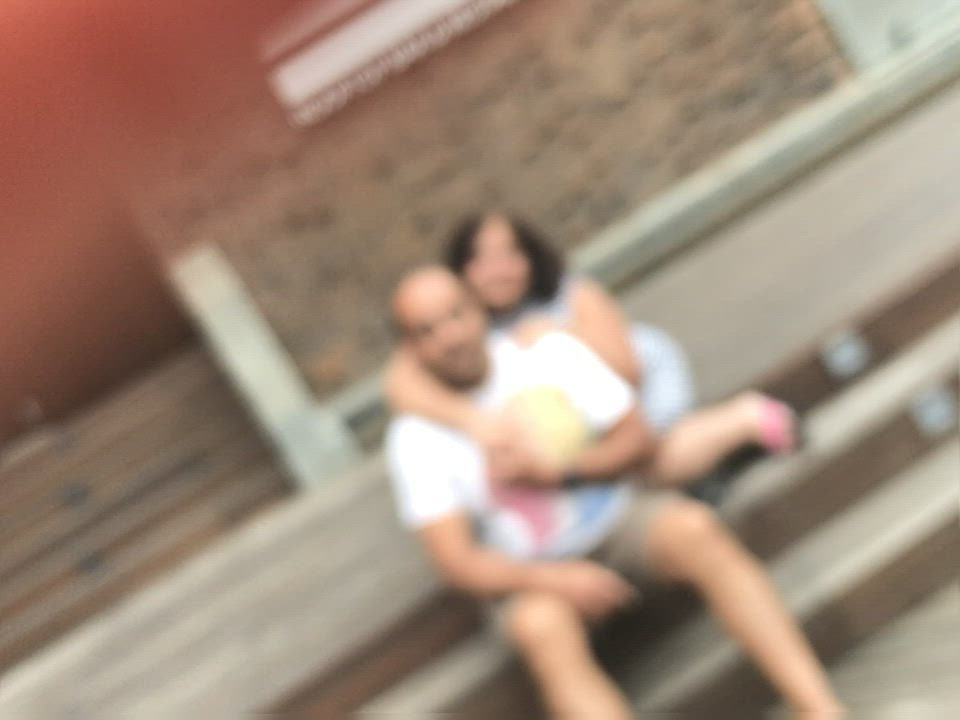In this blurry photograph, two African-American individuals are sitting on a set of three steps, with their pose creating an intimate and affectionate atmosphere. The man, who appears to be bald and is wearing a white t-shirt, is seated on the second step. Positioned slightly behind him, the woman, with her black hair cascading down, embraces him warmly. Her right arm drapes over his neck and shoulder, while her left arm wraps around him, her hands meeting in a tender clasp. The composition and their expressions suggest a close and loving relationship, capturing a moment of connection despite the image's lack of sharpness.